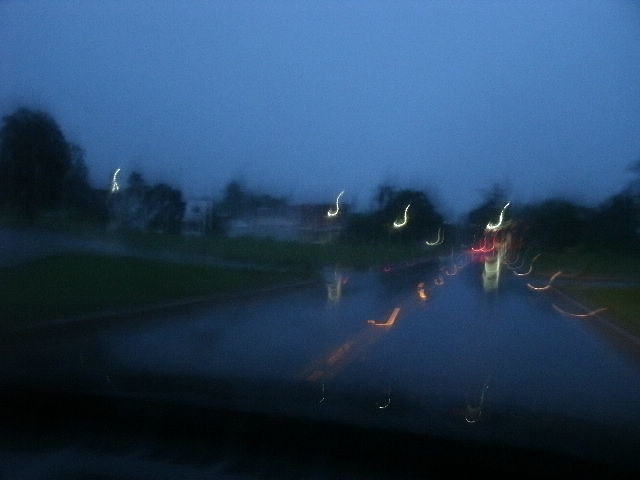Captured from a moving car during dusk, this photograph exhibits a high-exposure effect that transforms all light sources into elongated streaks, creating a dynamic and somewhat surreal visual. The street lights and reflections on the wet pavement form mesmerizing S-shaped patterns across the road, which is centered by orange lines stretching into the distance. In the background, elongated lights, likely from street lamps, add to the ethereal feel. On the left side of the image, a white house stands out against the darkening, deep blue sky, while patches of grass line both sides of the road. Shadowy trees loom in the distance, completing this atmospheric night scene that balances between clarity and blurred motion.